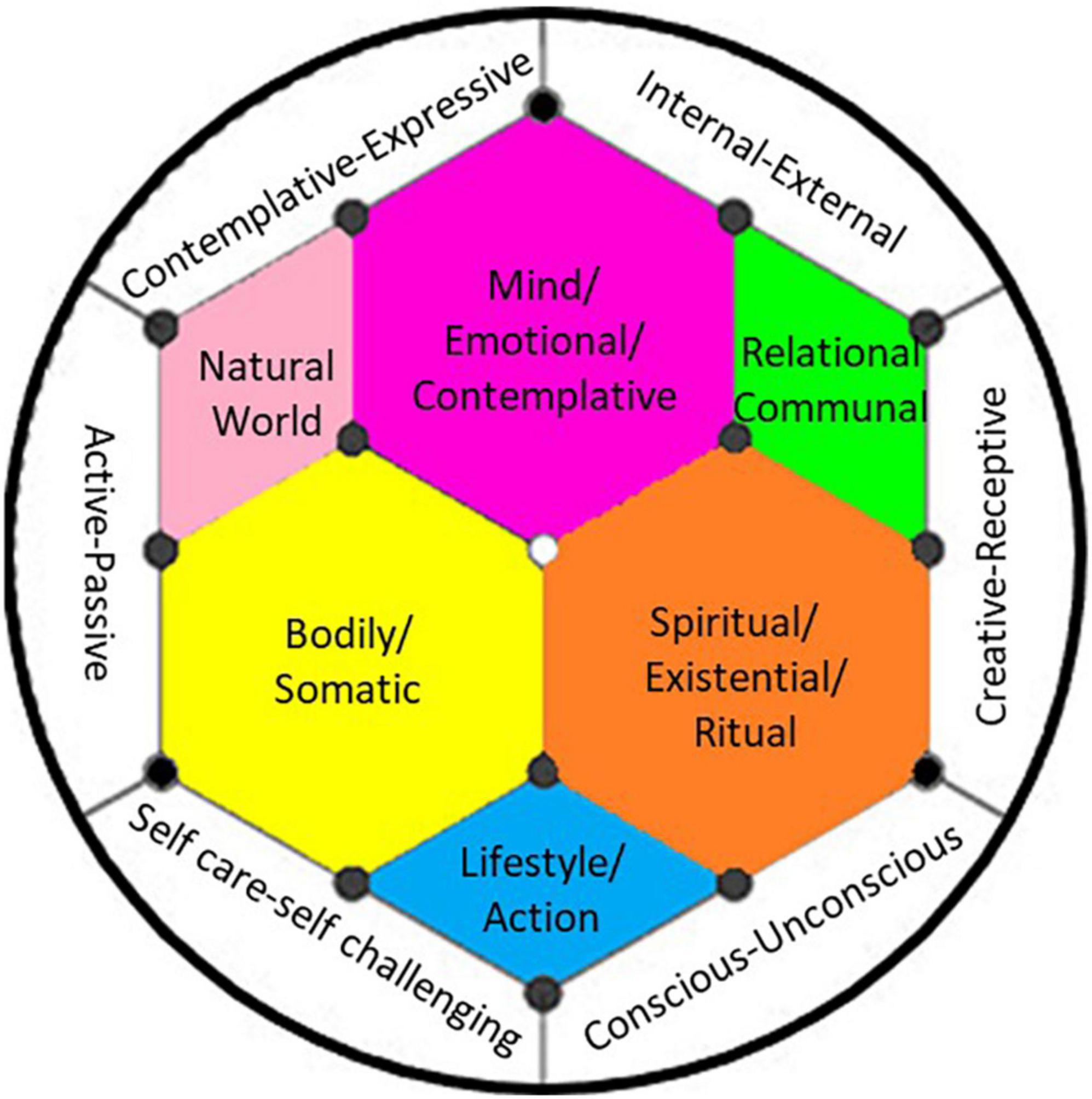This image appears to be a detailed diagram from a psychology textbook. The overall structure is a circle comprising an intricate hexagonal pattern and various colorful segments, resembling a soccer ball. The outer circle is divided into six sections, each containing paired terms: “Contemplative/Expressive” (top left), “Internal/External” (top right), “Creative/Receptive” (right), “Conscious/Unconscious” (bottom right), “Self-care/Self-challenging” (bottom left), and “Active/Passive” (left).

At the center, there are six distinct, color-coded divisions each denoting different aspects:
1. **Natural World** – Located on the upper left, shaded in light pink.
2. **Mind, Emotional, Contemplative** – Positioned at the top center, highlighted in bright pink.
3. **Relational, Communal** – Found at the upper right, marked in neon green.
4. **Spiritual, Existential, Ritual** – Situated at the bottom right, in orange.
5. **Bodily, Somatic** – Located at the bottom left, shaded in yellow.
6. **Lifestyle, Action** – Placed at the bottom center, represented in blue.

The diagram’s central hexagon is interconnected through black lines featuring black dots with white centers, which connect to different parts, predominantly parallelograms and diamonds, containing the text. This rich graphical representation uses vivid colors and shapes to categorize various psychological and relational attributes, emphasizing their interconnectedness.